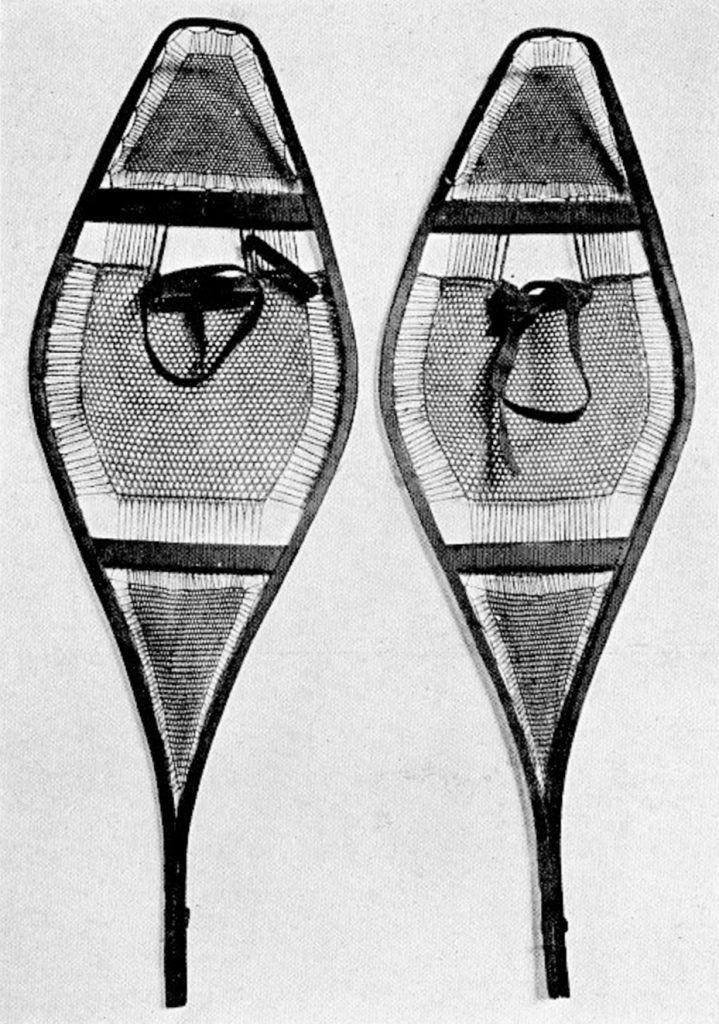The black-and-white photographic image showcases an overhead view of two traditional snowshoes, set against a stark white background. These old-style snowshoes are crafted from wood and feature intricate webbing made of twine and cloth bands for securing the feet. The snowshoes have a distinctive shape that expands from a narrow, pointed bottom to a rounded, diamond-esque top. The front of each snowshoe displays a prominent dark triangular or pyramidal structure, followed by a band and a middle section characterized by octagonal webbing where the feet would be placed. Near the tips, there is another band and inverted triangles of webbing. Lined up closely side-by-side, yet not touching, the snowshoes resemble paddles or tennis rackets and exhibit detailed craftsmanship designed for walking on snow.